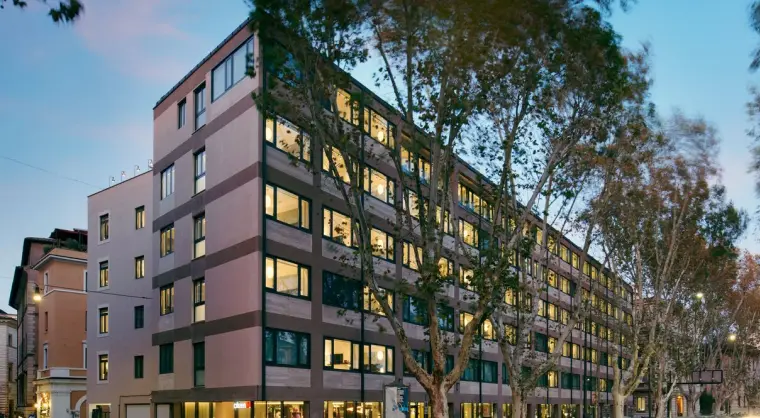The image is a highly detailed digital rendering, possibly from a video game, depicting a modernist six-story building. The building's design suggests it could serve as both retail on the bottom floor and office space on the upper five floors. Its architecture is characterized by a minimalist style with a palette dominated by browns and tans, accented by black window frames. The windows are large and aligned in a regular sequence. In front of the building, there is a row of trees, their dark green leaves offering a sharp contrast against the bright blue sky. The perspective seems to be from a slightly elevated position, giving a view that includes the tops of the trees, hinting at an urban environment where such trees might be planted along a median strip separating two lanes of traffic.